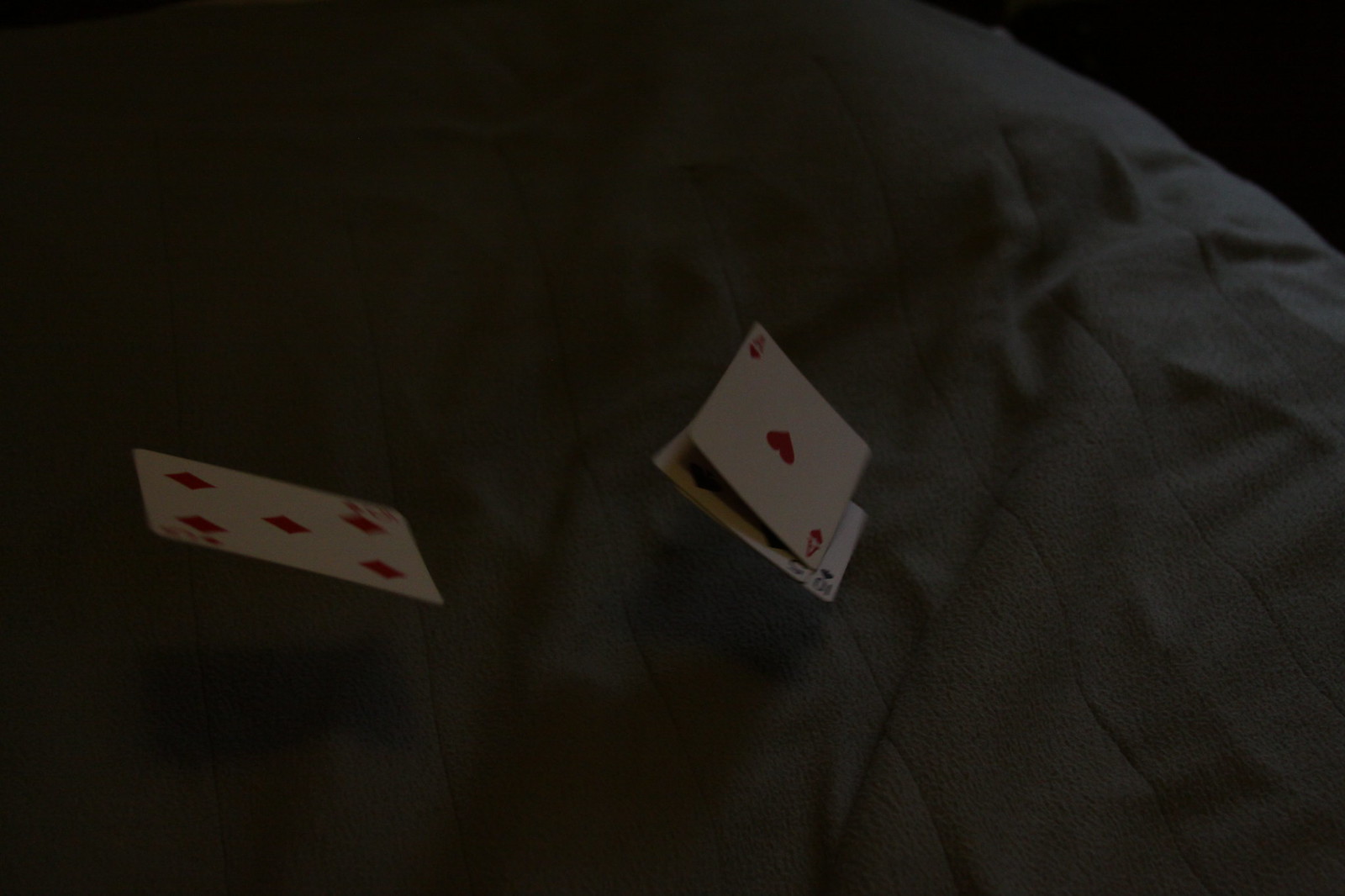In this image, a large, dark rectangle forms the backdrop, creating a somber and enigmatic atmosphere. The background is completely black, making it difficult to discern any additional features. Dominating the center of the picture is a gray blanket with visible lines running through its fabric. The blanket is characterized by its wrinkles and creases, which indicate it is folded in multiple spots. The exact boundaries of the blanket are not visible, as it extends beyond the edges of the frame.

Resting on this blanket are four playing cards, which are partially obscured and scattered across the fabric. Starting from the left, the first card is a blurry three of diamonds. To the right of the three of diamonds is an ace of hearts, followed by a five of spades. Slightly below and to the right of the ace of hearts is a ten of spades. The arrangement and partial view of the cards add to the mysterious and slightly chaotic feel of the photograph.